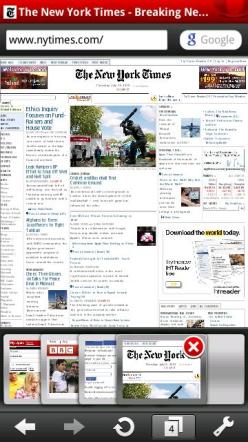A photo depicts an old smartphone, potentially one of the original iPhones or an early Android device, displaying the New York Times website. This device appears quite antiquated, evident from the visible Google search bar at the top and the desktop version of the New York Times website shown below it, reflective of a time before mobile-optimized websites were common. The screen features a header reading "New York Times," and in the search bar below, it reads "NewYorkTimes.com." At the bottom, there are four tabs likely indicating other news sources such as the BBC, along with two other indistinguishable sites. The navigation bar includes back and forward buttons, a refresh button, a tabs button, and a prominent settings button. The website's appearance is cluttered and disorganized, suggesting it predates modern standardized web design practices.